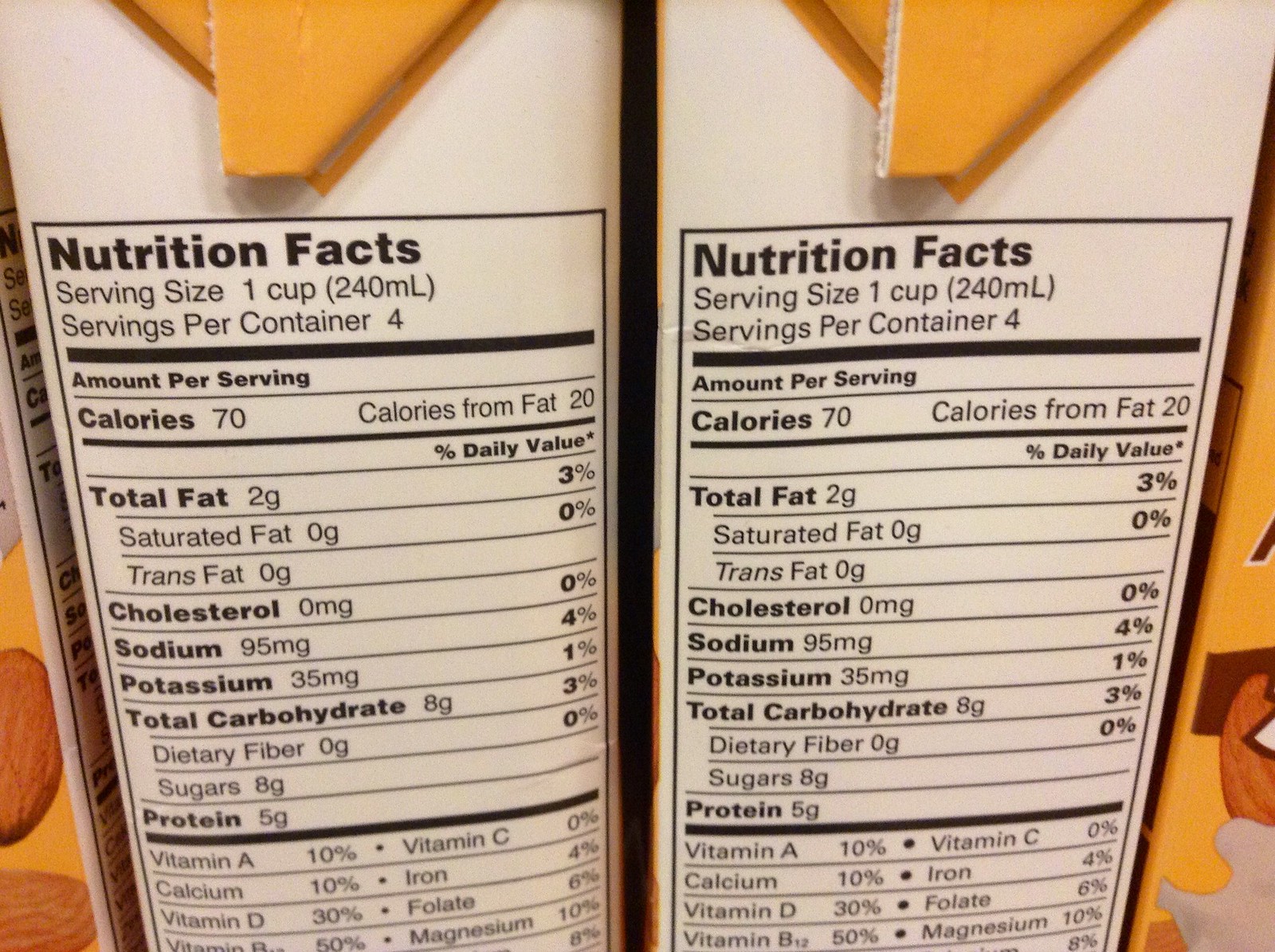This color photograph features the side-by-side Nutrition Facts panels of two identical shelf-stable cartons, both a grayish-white hue with a contrasting orange tip. The vibrant orange color is also partially visible on the far left and right sides of the image, hinting at the presence of additional cartons. On the front of these cartons, barely discernible, is a brown image. The prominently displayed Nutrition Facts reveal that a one-cup serving contains 70 calories, 2 grams of fat, 95 milligrams of sodium, 8 grams of carbohydrates, 8 grams of sugars, and 5 grams of protein.